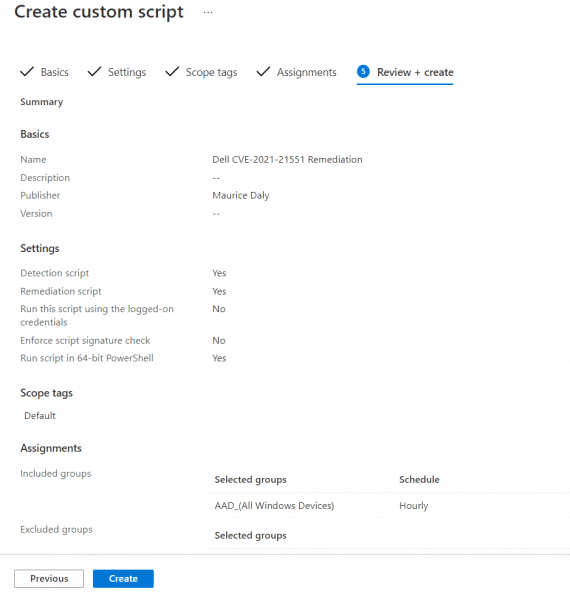The image depicts the "Create Custom Script" page of a software interface. At the top left corner, "Create Custom Script" is prominently displayed in black font. Below this title are five navigational tabs, each representing one of the sequential steps required to create a custom script. These steps are: Basics, Settings, Scope Tags, Assignments, and Review + Create. The final tab, Review + Create, is currently selected, as indicated by a thin blue bar underneath it.

The main section of the image is divided into multiple subsections, each outlined with detailed, structured information. 

1. **Basics**: This section includes fields for the Name, Description, Publisher, and Version of the script.

2. **Settings**: This section provides options for configuring various script parameters:
   - Detection Script: Yes
   - Mediation Script: Yes
   - Run the script using the log-on credentials: No
   - Enforce script signature check: No
   - Run script in 64-bit PowerShell: Yes

At the bottom of the Review + Create section, a summary is displayed consolidating all the choices made across the different steps. The summarized details include the script's basics as well as the settings configured in the previous steps.